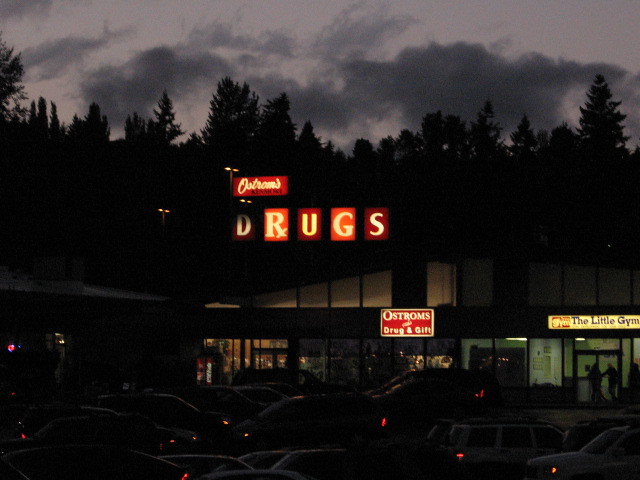A horizontal, rectangular night-time scene features a vintage shopping center with a prominent drugstore. In the middle of the image, a large red sign with varying shades of red letters spells out "Ostrom's Drugs," with the "D" less illuminated than the other letters. Directly below, another red sign with white lettering reads "Ostrom's Drug and Gift." To the right, a smaller, white rectangular sign, also with blue font, says "The Little Gym." Several cars occupy the parking lot, with their brake lights glowing red, casting a vibrant contrast against the dark environment. The sky above, shades of dusk with dark clouds, adds to the moody atmosphere. In the background, the dark shapes of tall trees outline the horizon. Two figures can be seen entering or leaving "The Little Gym," adding a touch of life to the otherwise quiet scene. The building has a low, triangular shape, indicated by the angling of the vertical windows with black panes.